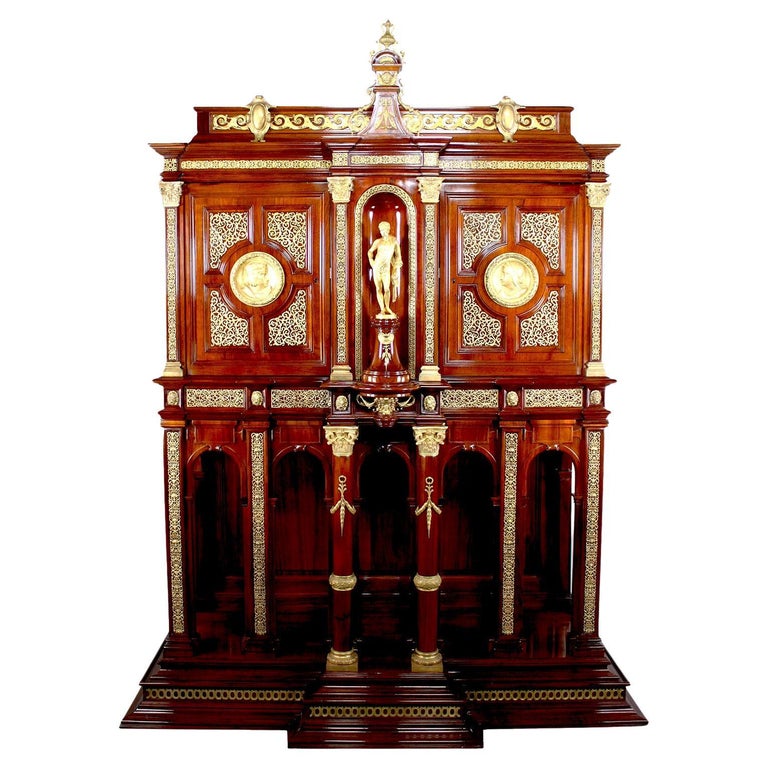This vertical image captures an intricate and elaborate wooden structure that resembles a miniature facade of a neoclassical building or an elaborate piece of furniture. The base is crafted from dark wood, leading up to two tiers of ornate design. 

The upper section features two cabinet doors with glass panels flanking a central alcove, which houses a gold statue of a man in a Greco-Roman style. Surrounding the statue and the upper tier are intricate gold decorative elements that frame the alcove and extend to an elaborate roof above it. 

Below, the lower tier is composed of an open area supported by six columns: four smaller pillars in the back and two larger, more elaborate pillars in the front, each adorned with gold trim and positioned on small pedestals. To the sides of this tier, there are gold pendants resembling heads embedded in the walls. The overall craftsmanship and detail, including the use of gold and the multiple classical elements, suggest that this piece could be an artistic representation of an ornate, neoclassical building or a complex mechanical clock without visible mechanics.